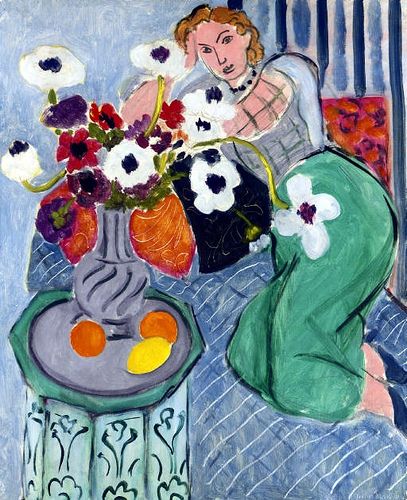This painting by Henri Matisse, titled "Harmony in Blue," features a woman reclining on a blue chaise lounge. She has shoulder-length red hair and fair skin, with a contemplative expression as she gazes towards the artist. The woman is dressed in a gray and blue top paired with a muted green skirt, complementing the overall blue and gray tones of the artwork. She reclines against a red pillow with purple flowers and a contrasting black pillow with a white flower, her right side resting on the chaise. Her right hand supports her head, and her left arm is crossed in front of her, adding to her relaxed pose.

In the foreground, a small round teal table holds a gray vase brimming with a vibrant bouquet: eight large white flowers with purple or black centers, as well as several red and dark purple blooms. Beside the vase are two oranges and a lemon, adding a splash of citrus color. The background is a harmonious blend of blue shades, featuring an orange and purple square behind the woman's head, with alternating light and dark blue stripes on the wall. The careful coordination of blue and green hues, combined with the subtle interplay of other colors, encapsulates Matisse's mastery in creating a serene yet dynamic composition.